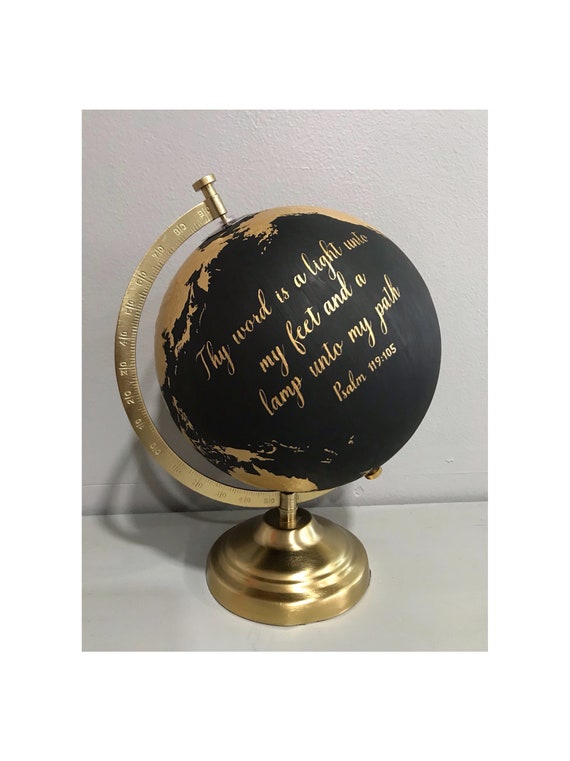The image captures an artistic photograph of a decorative globe, prominently positioned on a white tabletop, with a white wall serving as the backdrop. The globe is mounted on a brass stand featuring a circular compass design, complete with a semi-circular, C-shaped arm that allows the globe to be tilted and spun. The base and arm of the stand are brushed in gold, and the arm is etched with ruler-like lines and measurements for a touch of detail.

The globe itself deviates from traditional earth tones, being painted in matte black to represent the oceans, while the continents and islands are elegantly highlighted in gold. Overlaying a large section of the Pacific Ocean, a Bible verse is inscribed in gold script, reading, "Thy word is a lamp unto my feet and a light unto my path," from Psalm 119:105. This artistic piece melds functionality with spiritual significance, creating an eye-catching and meaningful decorative object.